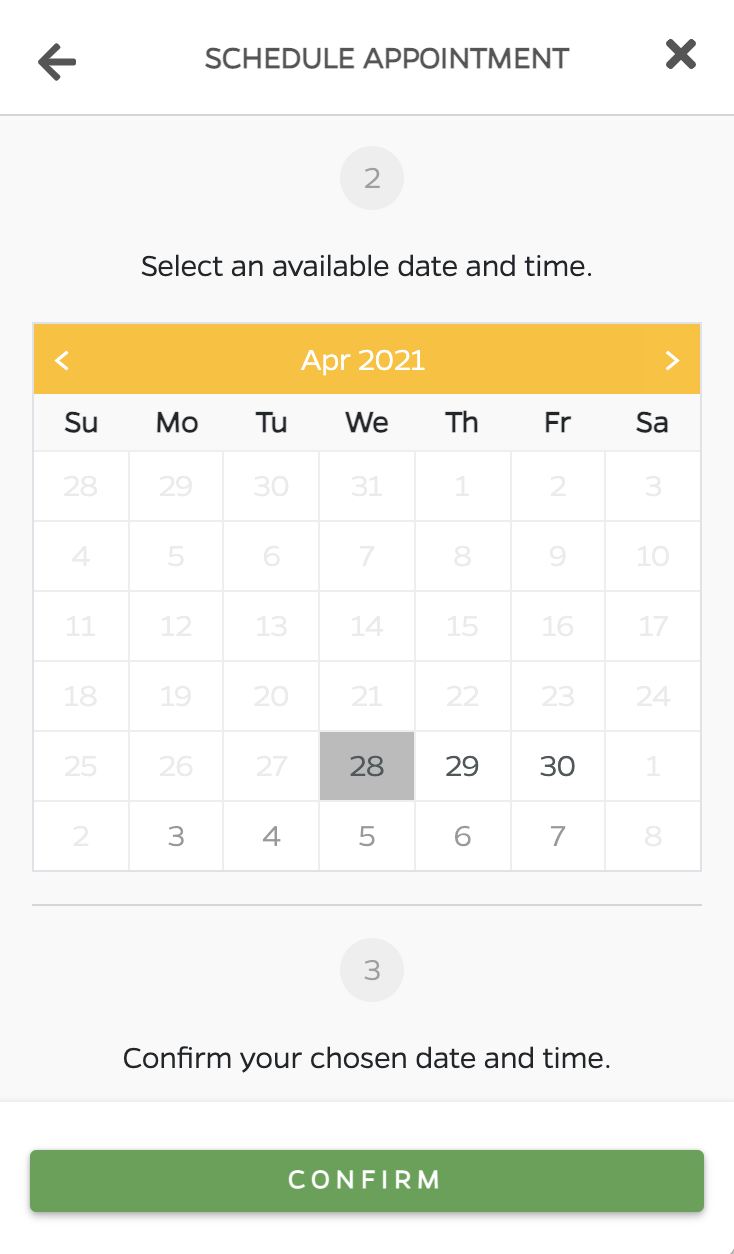A mobile screenshot detailing the process of scheduling an appointment. The page is primarily white with black text, except for a green confirmation button at the bottom. At the top, there's guidance labeled "How-to: Schedule an Appointment." The visible content seems to be divided into instructional steps. 

The first step is to select an available date, represented by a calendar displaying the end of April 2021. The available dates are specifically the 28th, 29th, and 30th of April.

The next part of the process instructs you to confirm your chosen date and time. This confirmation can be completed without the need for a phone call, suggesting the entire process is virtual. The green 'Confirm' button at the bottom of the page highlights the final step to finalize the appointment.